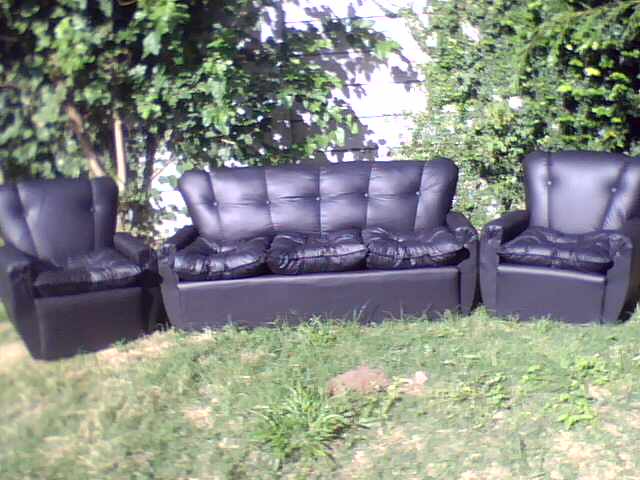In the photograph, there is a set of three black leather or faux leather furniture pieces arranged on a lawn during a bright sunny day. The set consists of a three-seater sofa positioned in the center and flanked by two matching love seats, one on each side. All three pieces feature tufted seat and back cushions. The seat cushions on both the sofa and love seats appear worn, with some cushions showing discoloration and a shriveled texture, indicating possible damage or spills. The grassy lawn on which they sit is mostly green but has patches of yellow and brown grass and dirt in some areas. Behind the furniture, the scene includes a backdrop of small shrubs and trees that cast shadows against a white wall or fence with horizontal slats. The image appears slightly blurry, adding a sense of age or wear to the scene, which might suggest that the furniture is being showcased for a sale.